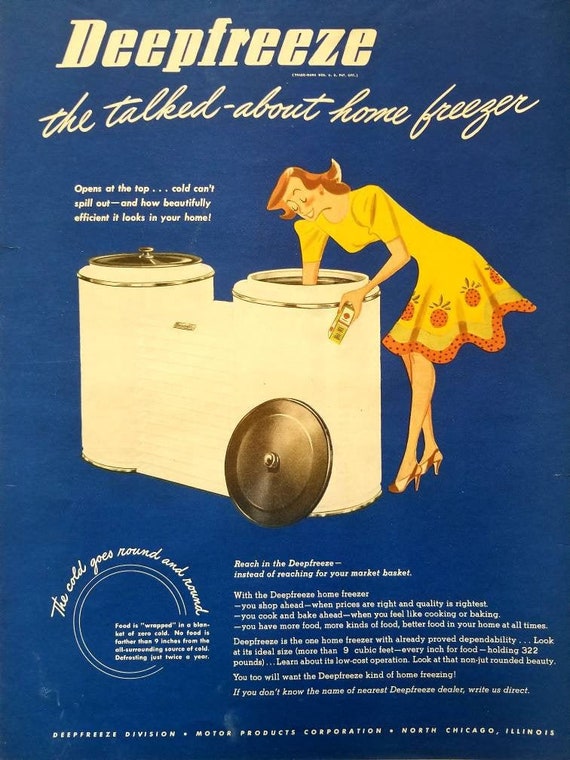This vintage advertisement from the 1950s promotes the "Deep Freeze," a heavily discussed home freezer of the era. The ad features a stylish retro design with a catchy caption at the top that reads "Deep Freeze, the talked about home freezer." The advertisement is set against a royal blue background with bold red lettering. A cheerful woman, adorned in a yellow dress with orange pineapple prints and high heels, bends over with a smile, reaching into the twin-cylinder deep freezer, her curly brown hair adding to the 50s aesthetic.

The innovative freezer offers two connected sections, each with its own lid that opens from the top, ensuring that the cold air doesn't spill out. The text emphasizes the freezer's efficiency and visual appeal in the home, highlighting the convenience of "reaching in the deep freeze" instead of always shopping. It boasts a spacious nine cubic feet capacity and promises a "blanket of cold" that keeps food well-preserved. The bottom of the ad is packed with additional information about the freezer, extolling its advantages for meal planning and food storage. The advertisement is from the Deep Freeze division of Motor Products Corporation, North Chicago, Illinois.